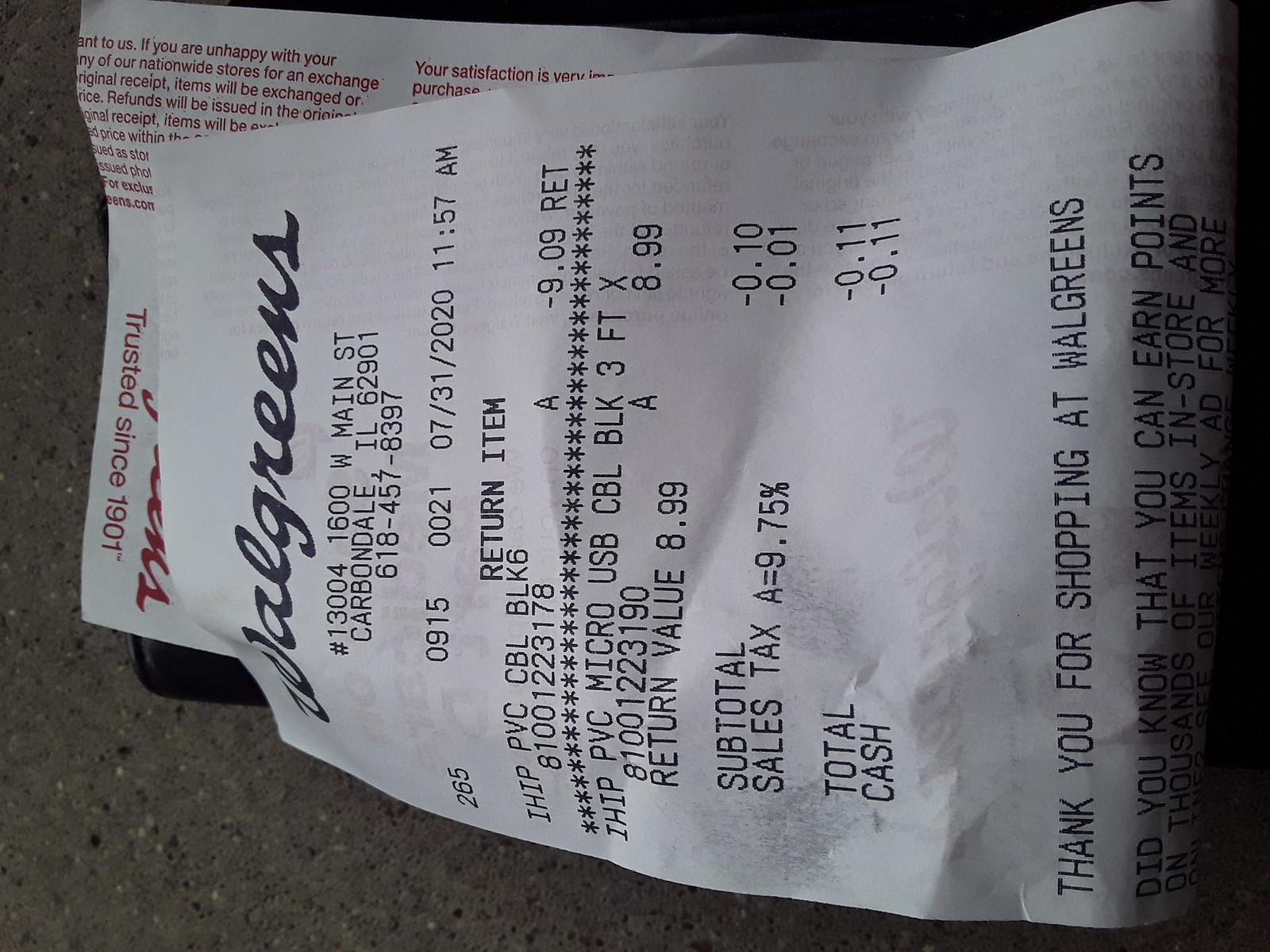In this image, a gray tabletop serves as the backdrop for a slightly wrinkled, white receipt from Walgreens. The receipt, displaying black ink, reads "Walgreens, number 13004, 1600 West Main Street, Carbondale, Illinois, 62901," and includes the store's phone number. It itemizes a return transaction for an item priced at 10 cents with an additional 1 cent tax, amounting to a total refund of 11 cents. The receipt also expresses gratitude with a message that says, "Thank you for shopping at Walgreens." Additionally, the receipt is folded over, revealing a glimpse of red writing on the back.